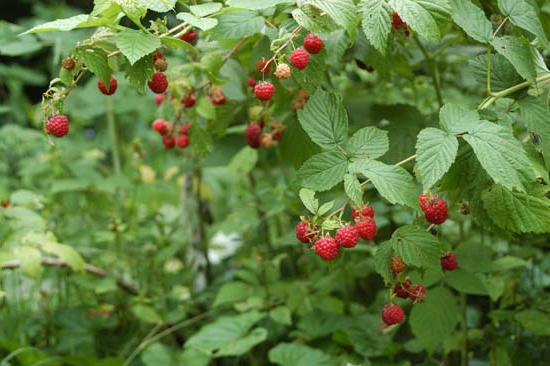In this image, we see a dense raspberry bush, likely situated in the wilderness. The scene is filled with lush green vegetation and small, flat leaves with a scissor-like appearance, lacking actual spikes. Several branches, especially from the upper right, hang heavy with raspberries of varying ripeness. The berries range in color from unripe whites and greens to fully mature, deep reds. There are about 30 berries in total, displaying the characteristic circular bumps that form round, clustered fruits typical of raspberries, although they might be slightly denser and more tightly packed together. The vivid contrast between the rich reds of the ripe berries and the lighter hues of the unripe ones adds to the natural beauty of the scene.